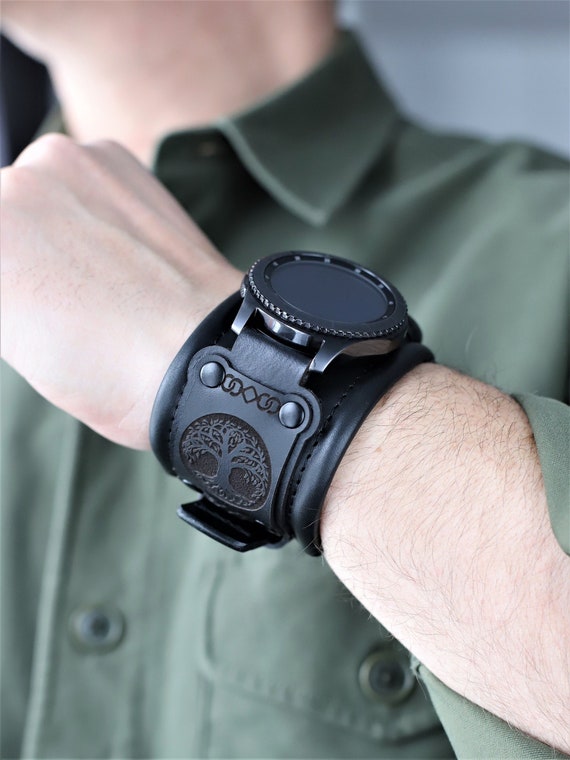This photograph is a close-up of a young man's chest and neck, which are slightly out of focus in the background, while his left forearm and hand are sharply in focus in the foreground. The man, of European descent, is wearing a medium to army green long-sleeve shirt, which is slightly unbuttoned at the collar. The shirt appears somewhat grayish green, giving a neutral tone. His arm is clenched, displaying a wristwatch with a prominent, wide black leather band, approximately two to three inches in width. The band features two black metal buttons and intricate burnt engravings, including a circular design and a tree with branches that span the width of the band. The watch face is black metal with a glass cover that has a textured, ribbed edge. The man gazes towards the left side of the photo, adding to the focused display of the detailed and personalized watch.